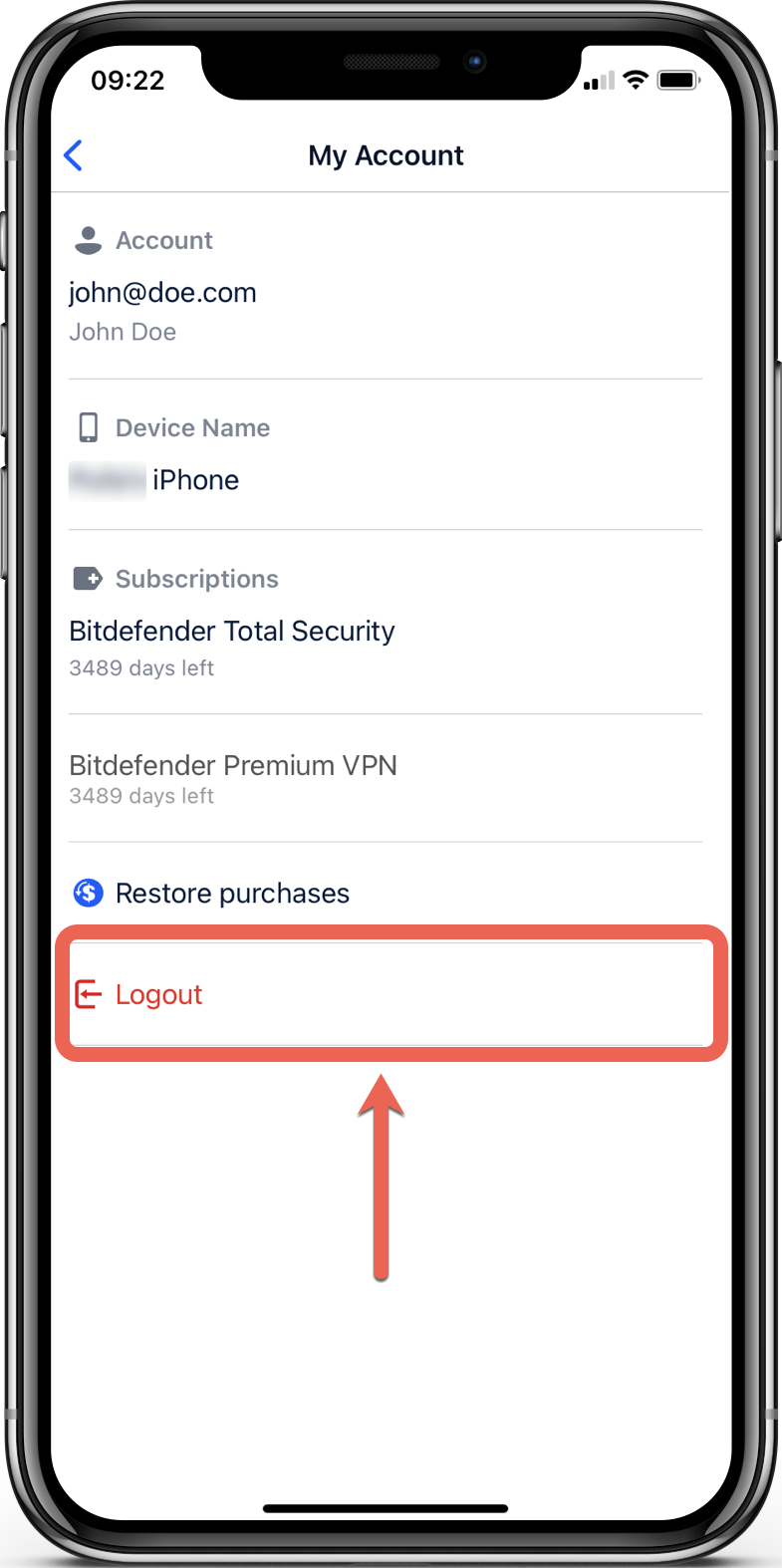The image depicts the front screen of an iPhone, focused on the 'My Account' settings page. The device has a dark silver edge, providing a sleek contrast to the white background of the screen. 

At the top left corner, there is a blue arrow pointing to the left. Immediately below it, the page title 'Account' is displayed, followed by the account email address and name. The next section labeled 'Device' shows the name of the iPhone, which has been pixelated for privacy.

Following this is the 'Subscriptions' section. Here, two subscription entries are visible: 'Bitdefender Security' with 3,489 days remaining, and 'Bitdefender Premium VPN' also with 3,489 days remaining.

Further down, there is an option to 'Restore Purchases,' and at the very bottom is a red-outlined rectangle with the word 'Log Out' inside it. An arrow in the center of the screen points directly to this rectangle, indicating that it's the button to click to log out.